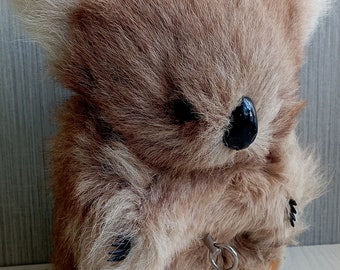This detailed photograph showcases an aged stuffed koala bear set against a gray pinstripe wall and placed on a cream-colored floor. The close-up image displays primarily the koala's face and belly. The fur transitions from a dark brown to a tan and finally to an almost white, giving a worn, matted appearance, hinting at the stuffed animal's age. A tiny white-edged ear is partially visible, adding to the lifelike detail. The koala's prominent features include a shiny, black plastic nose and small, round black eyes. The front paws, which resemble stylized black felt pieces, peek out from beneath the fur, revealing their toy-like nature. Additionally, there appears to be a key or key ring in the middle of the koala's chest, suggesting it may have been a musical or talking toy, or perhaps used as a backpack accessory. Despite its years, the koala’s stern, almost menacing expression is unmistakable, emphasizing its character as a beloved but strict-looking stuffed animal.